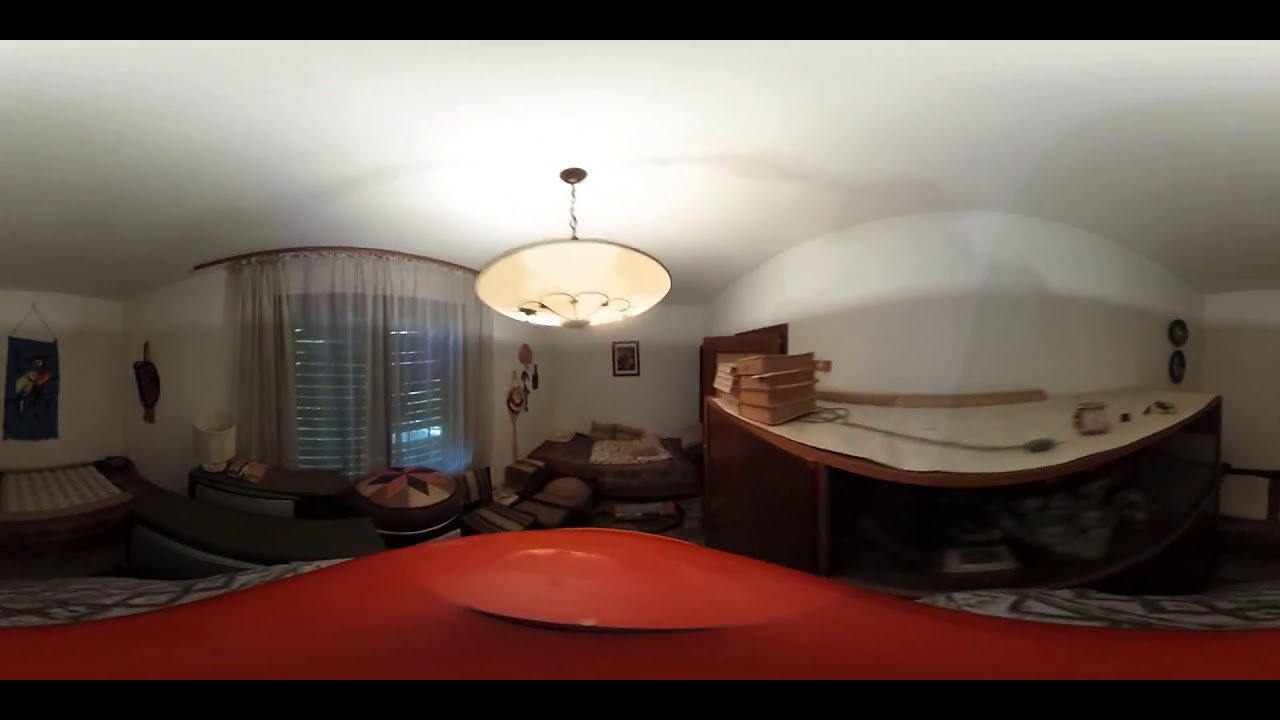This is a panoramic photograph of a spacious living room that appears slightly distorted due to a fisheye effect, giving it a curved appearance. The walls and ceiling are painted white, and the room is furnished with an array of items. In the center hangs a semi-circular chandelier decorated with heart designs. To the right, a rounded desk stocked with thick files and books catches the eye, next to what looks like a pool table or another desk, though it appears stretched. The focal point includes a large red area and a green-and-white rug at the bottom of the image, likely leading to an ottoman. A couch adorned with a blanket sits comfortably within the room. The windows to the left are curved, with cream-colored curtains and blinds that are drawn. Natural daylight filters through, casting light onto a side table and a bench. The walls are also adorned with several paintings and photographs, adding a personal touch to the room's aesthetic.